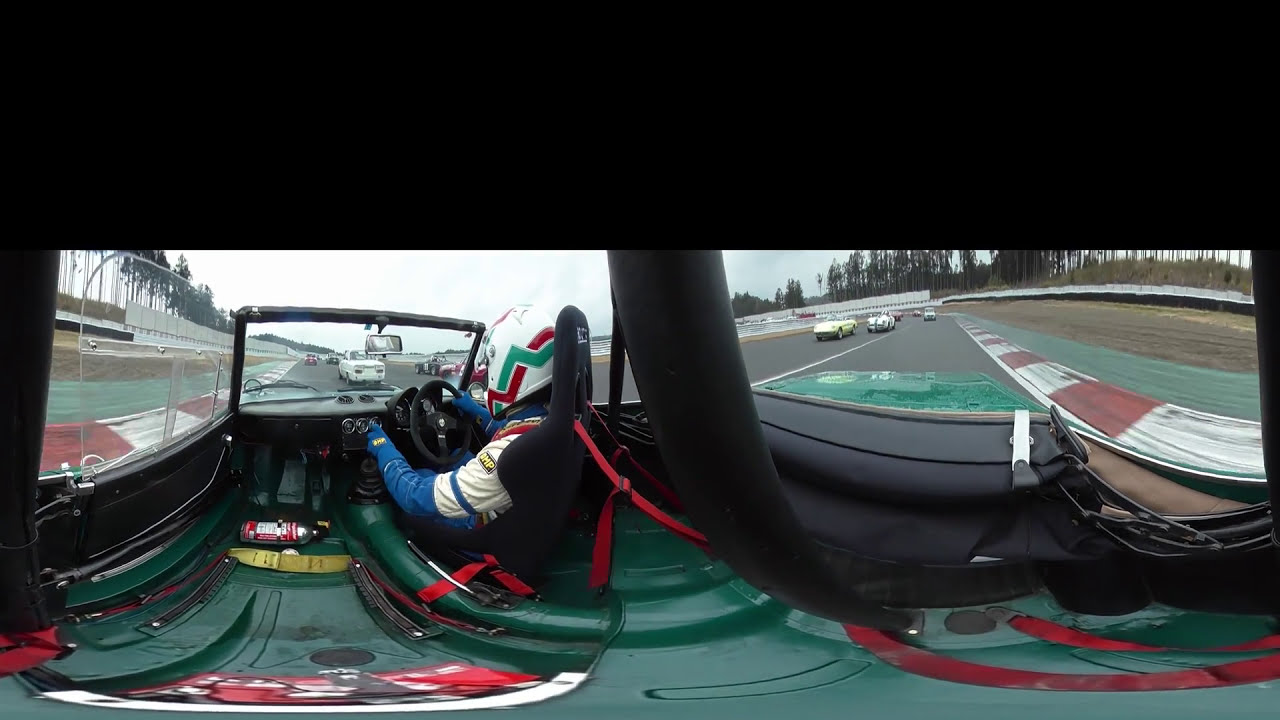In this image, we see a wide-lens view, potentially a screenshot from a video, capturing a vibrant scene on a race track. Centrally positioned, a race car driver is seen from behind, wearing a racing suit in white, blue, and red, along with a helmet that bears colors white, green, and red. The driver, inside a green, Jeep-like convertible with a roll cage, grips the steering wheel. The car's interior features red seatbelts and straps, as well as a silver tank on the floor adorned with a red label. A mix of black areas and windows accentuate the vehicle's design.

The racing track stretches out beneath a cloudy, gray sky, bordered by red and white lines and flanked by green grass and trees. Cars in white, yellow, black, and one with a blue stripe can be seen in the distance, adding to the dynamic atmosphere of this midday outdoor race. The top of the image has a black border, and no text is visible anywhere in the scene. This detailed snapshot encapsulates the intensity and vivid colors of a race day.